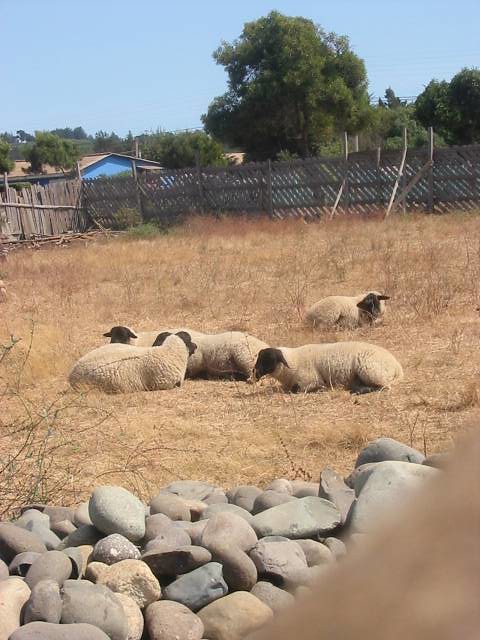In the foreground of the image, a cluster of gray and light brown rocks lay scattered on dry, wiry, yellow grass, interspersed with patches of straw and dirt. Nestled closely together in the center of the frame are four sheep, characterized by their off-white woolly bodies contrasted with black faces and ears, resting seemingly under the midday sun. These sheep are within a large pen bordered by a wooden slatted fence, which shows signs of aging and structural decline. Beyond the fence, the backdrop features a scenic mix of elements: an array of large, lush green trees, hints of a turquoise house with a gray roof, and a blue sky peeking through. The entire composition suggests a serene and somewhat rustic setting, possibly a quaint neighborhood or someone's expansive backyard.